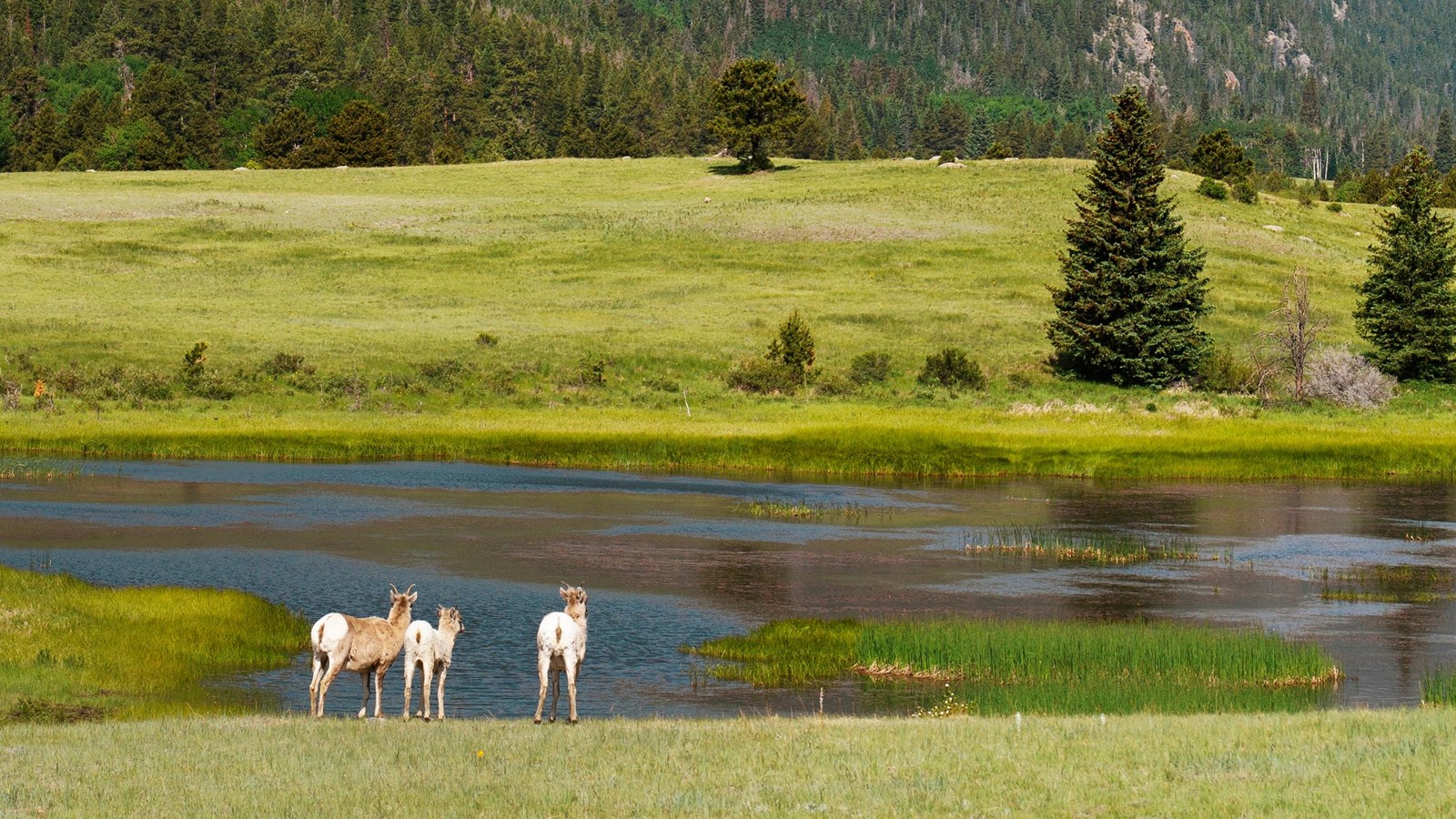In the image, three animals resembling llamas, potentially deer or antelopes with small backward-facing horns, stand in the lower left corner facing a body of water. These animals display a mix of brown and white colors. The water, possibly a river, shows clear blue stretches interspersed with green and brown areas influenced by aquatic vegetation. Sedges and grasses are visible in and around the river. The animals stand in a field of vibrant green grass leading to the water, surrounded by occasional evergreen trees with deep green foliage. Beyond the river, the landscape transitions into a gently hilly area with well-mowed grass and more trees, eventually giving way to a mountainous backdrop. These mountains feature a mix of evergreen forests and rocky outcrops, adding depth and diversity to the scenic view.